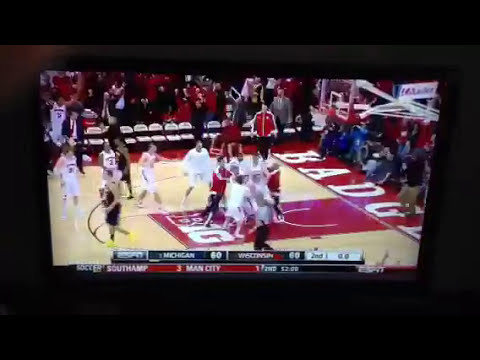This image depicts a slightly blurry, low-quality photograph of a flat-screen TV displaying a live college basketball game between Michigan and Wisconsin, with both teams tied at 60 points. The game appears to be in the second quarter with no time remaining, as indicated by the scoreboard on the screen. The court features light wood flooring with bright red accents, and players can be seen in white and red jerseys. On the right side of the court, several players are clustered together, likely contesting for the basketball. There are also players in black and white jerseys dispersed around the court. In the background, the seats for the crowd can be seen, as well as the mostly empty benches for the teams. The image appears to have been captured in a dimly lit room, emphasizing the light from the TV screen. An additional TV announcement is visible at the bottom of the screen, mentioning another match with "Southam 3, Man City 1" and "12 minutes left."